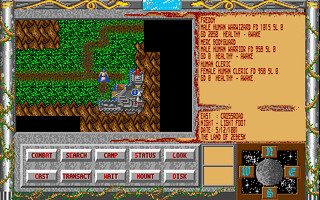This screenshot from a retro video game, reminiscent of graphics from the 80s or 90s, features a pixelated, isometric interface. The main view shows an armored adventurer traveling along a dirt path flanked by grass. Below the scene, there are gameplay buttons labeled "Combat," "Search," "Camp," and "Status." The image is rich with details, including a small rectangle depicting a silver pole adorned with yellow ribbons and green flowers. A compass with directions marked N, E, S, W is located at the bottom right. The upper left corner shows a green background and a tiny soldier figure, while the top right corner contains partially readable text, likely indicating character information such as "Frieden male."